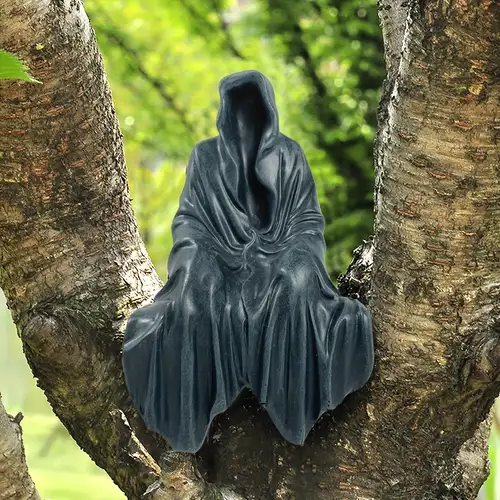In this image, we see a vibrant outdoor setting with lush, green trees and branches forming a backdrop under a bright sunny sky. At the center of the picture stands a tree trunk that splits into multiple branches, creating a U-shaped nook where a plastic figurine is perched. This figurine, resembling a Grim Reaper or a ghostly figure, is cloaked in a long, dark robe—a deep black or very dark gray—that conforms to the shape of an invisible body sitting with its hands on its knees. Notably, the hooded figure has no face, chest, or visible body parts, giving it an eerie, spectral appearance. Despite the realistic setting, the figure seems photoshop-enhanced, likely intended as a Halloween decoration, adding to the spooky ambiance of the scene. The cloak drapes naturally over the unseen form, intensifying the mystery of its presence amongst the lush greenery.